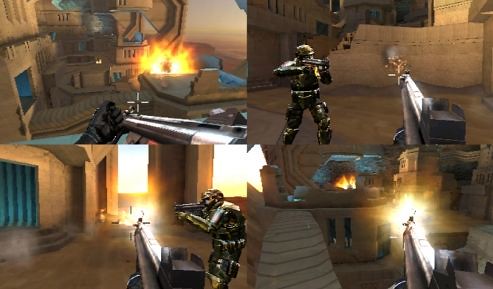The image is a computer-generated screenshot from a first-person shooter video game, divided into four distinct quadrants, each showing a different player's perspective. The background is dominated by a medieval-like village encased in brown stone buildings and pathways, resembling an old castle's interior. Players, visible in each section, are equipped with futuristic, robotic-looking armor akin to stormtrooper gear and are holding guns, some of which are mid-fire, producing red flare effects. Notably, in the top-left quadrant, one player is reloading their weapon, their black-gloved hand visible on the gun. The environment is interspersed with small windows and doorways, and there are elements of bright light and fire that add dynamic contrast to the otherwise earthy and metallic tones of the scene.